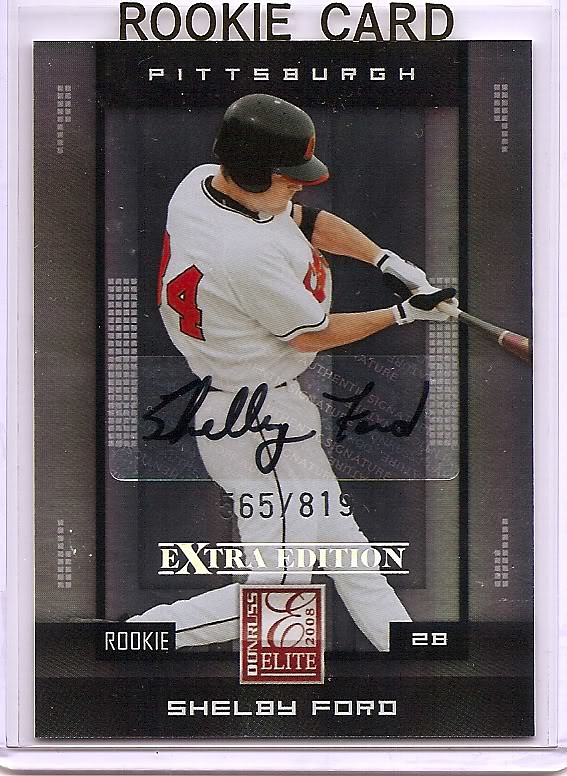The image showcases an autographed baseball card featuring Pittsburgh rookie Shelby Ford. Dominating the entirety of the image, the card's top reads "Rookie Card, Pittsburgh." Central to the card is an action shot of Shelby Ford mid-swing with a black baseball helmet over a red cap, adorned in a white jersey marked with the number 34 in red, accented with white stripes on the short sleeves. He wears white batting gloves with black thumbs, holding a black bat with a red tip and white grip, which slightly extends beyond the frame. The card displays Ford's signature centrally in black sharpie. Below, the text "565 out of 819, Extra Edition Rookie, 2B, Shelby Ford" and "Donruss Elite Cards 2008" imparts its collectible significance. The color scheme includes white, black, gray, silver, red, and orange accents, making it a valuable addition to any collection.